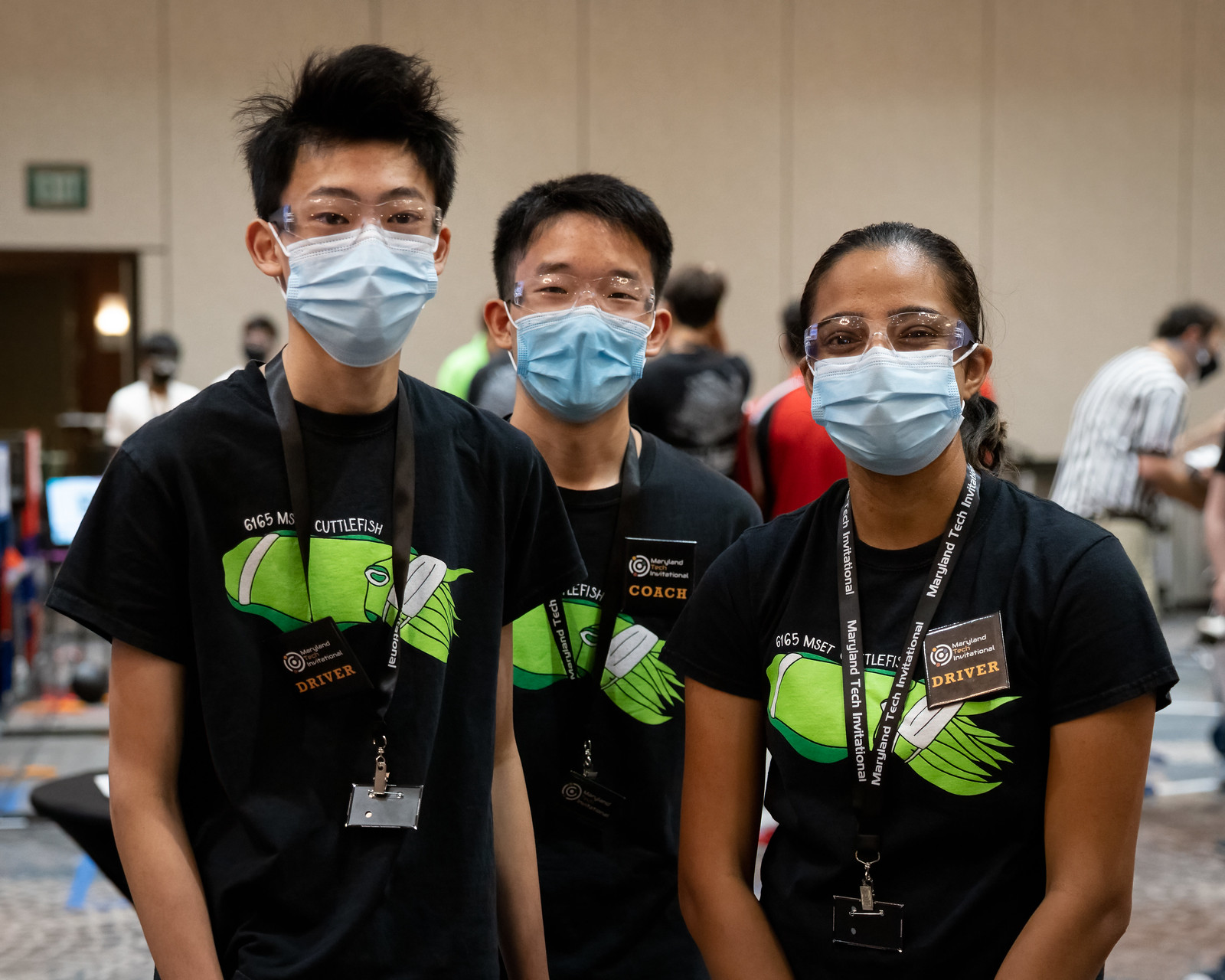The image features three young individuals, likely students, standing upright in a well-lit conference room with cream-colored walls, which could be a hotel or school conference room. There are people visible in the background, all wearing masks due to the COVID-19 pandemic. Each of the three youths wears a blue surgical mask, dark black short-sleeved t-shirts featuring a yellow and orange cuttlefish, which is also depicted wearing a mask, and matching lanyards with name badges. The young man on the left has dark hair and appears to be of Asian descent, as does the young man in the center, while the young woman on the right, who has slightly darker skin, wears clear protective glasses. All three individuals have glasses and seem to be smiling with their eyes.